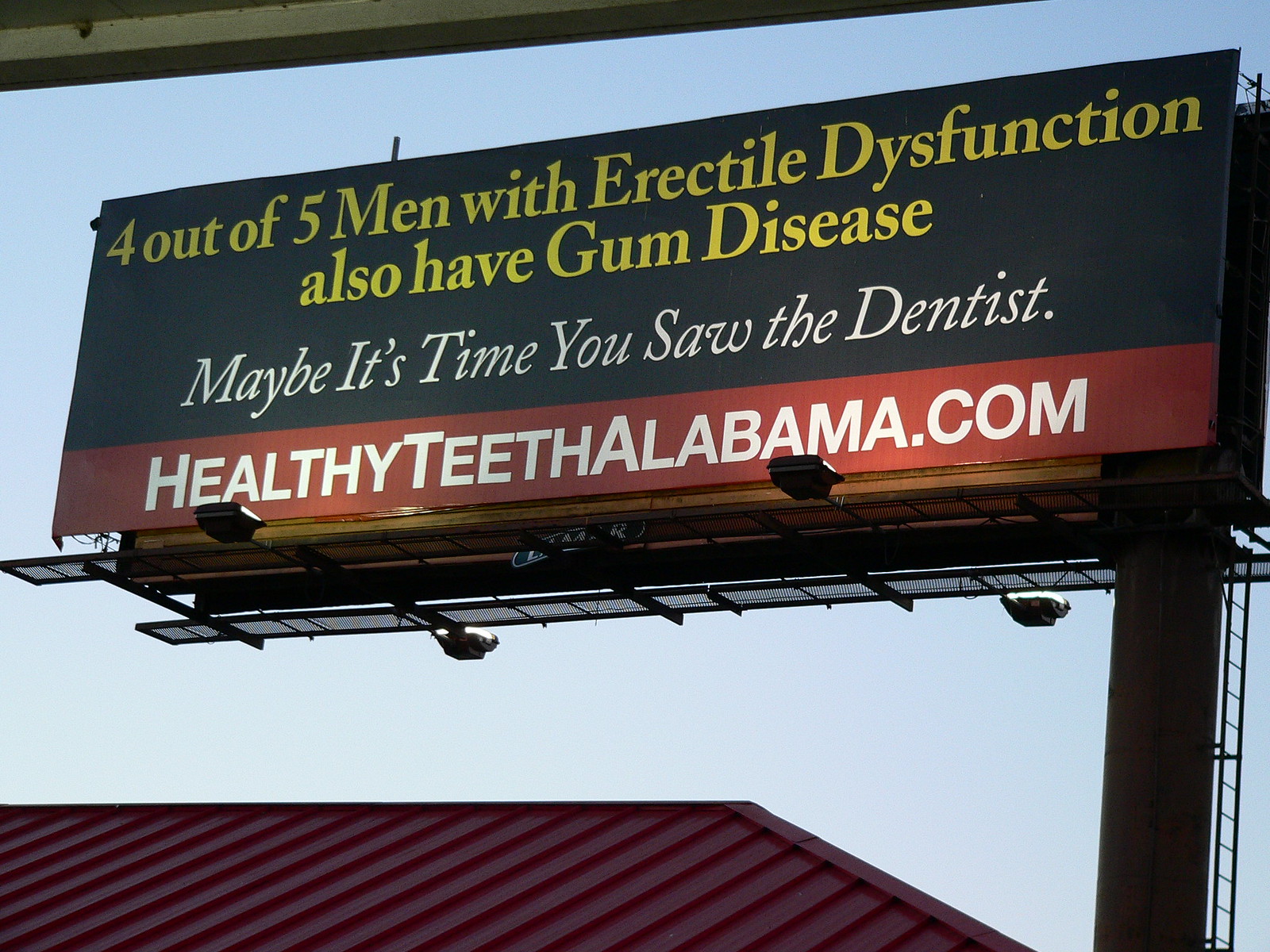The photograph captures a prominent billboard set against a vibrant blue sky on a clear daytime scene. The billboard itself features a stark black background and is illuminated by spotlights from below, ensuring its message stands out. The main text on the billboard is bold, informative, and somewhat provocative: "Four out of five men with erectile dysfunction also have gum disease," written in striking yellow text. Following this, in elegant italics, it reads, "Maybe it's time you saw the dentist." At the very bottom of the billboard, a red strip contains the text "healthyteethalabama.com" in white. 

The billboard is mounted on a sturdy pole, which also supports a ladder, presumably for maintenance purposes. The frame surrounding the billboard is black, complementing its overall aesthetic. Below the billboard, a red roof slightly intrudes into the frame, adding a splash of color to the composition. Above the main billboard, the very bottom portion of another billboard can be seen, though its text is illegible. The combination of a clear blue sky and strategic lighting makes the billboard's message both visible and impactful.